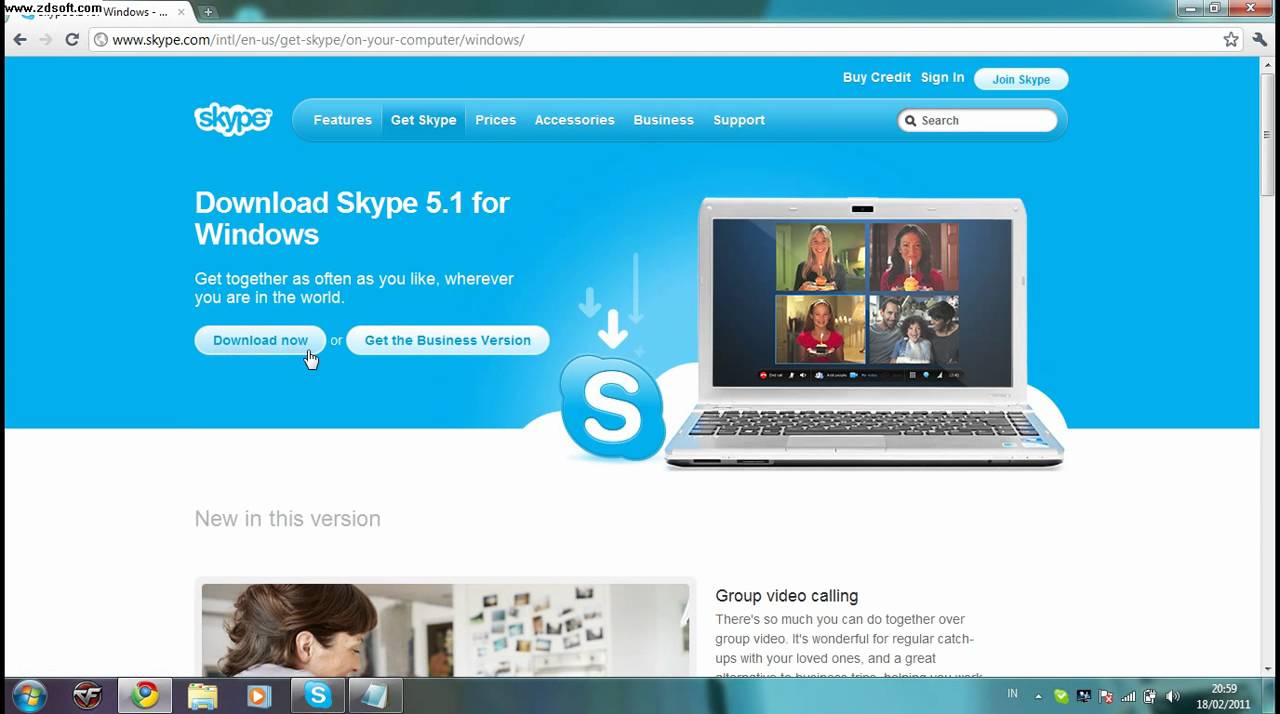The screenshot captures an antiquated version of the Skype homepage, prominently featuring the URL "Skype.com" at the top. Central to the page is the Skype logo, beneath which a message reads: "Download Skype 5.1 for Windows. Get together as often as you like, wherever you are in the world." Below this message is an inviting blue button labeled "Download Now." Adjacent to this button is the option to either download the standard version or "Get the business version," emphasized by an "Or" placed between two buttons.

On the right side of the screenshot, there is a visual of a laptop displaying a video call in progress, featuring four individuals actively engaged in a Skype conversation. To the left of this image, the text "New Windows Version" stands out, followed by a brief description that elaborates on the features and benefits of the updated version. The overall layout exemplifies an early 2000s web design aesthetic, reflecting Skype's functionality and user-friendly focus from that era.